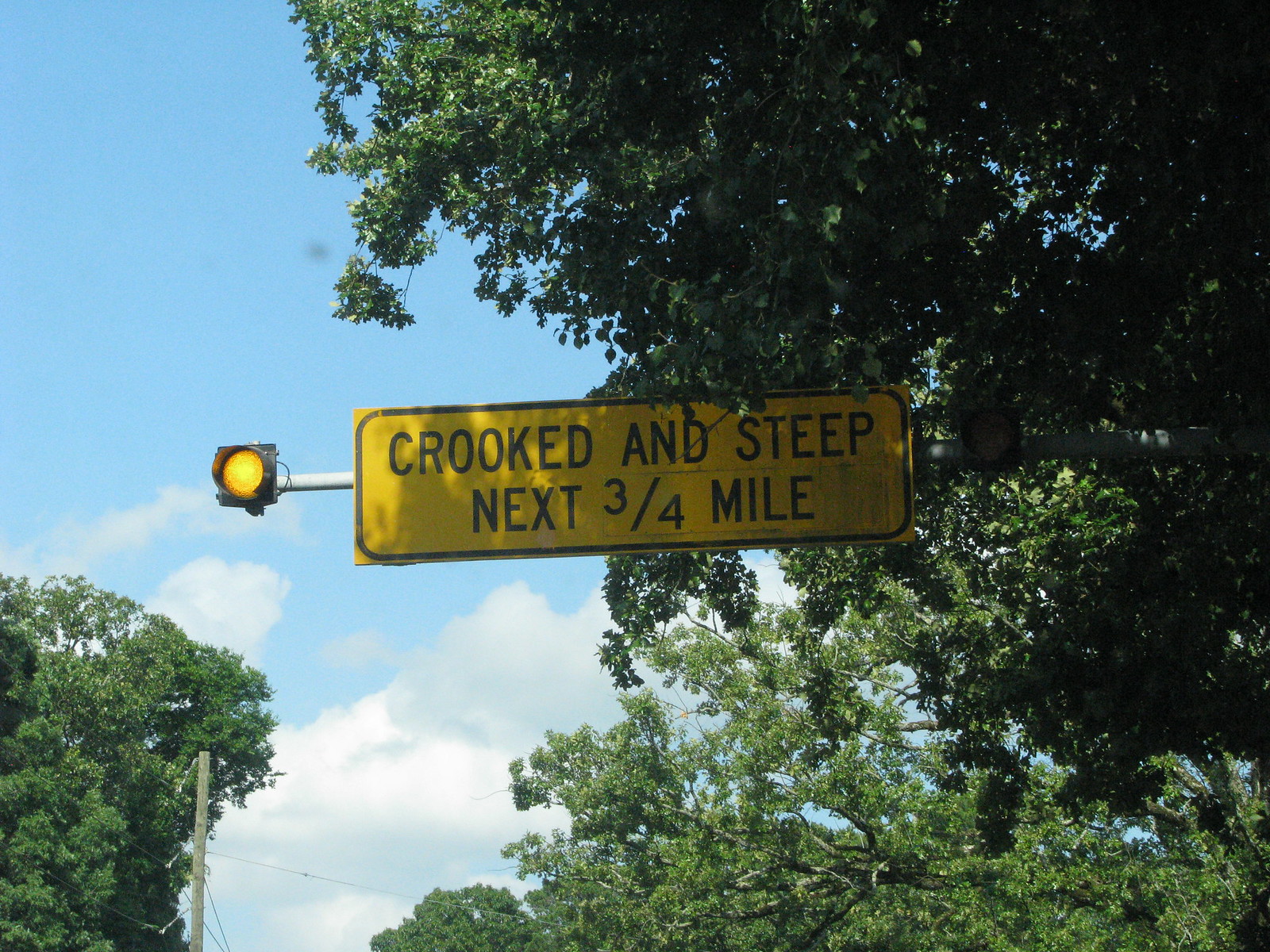The photograph captures a street scene focused on a cautionary road sign taken from below, likely from the perspective of someone standing on the road. Dominating the center of the image is a large rectangular yellow sign with a black border, featuring the text "CROOKED AND STEEP NEXT ¾ MILE" in bold capital letters. To the left of this sign, there is a single traffic light mounted on a horizontal, heavy metal crossbar typically found on wider, busier roads. The traffic light is illuminated in solid yellow, indicating caution. The background is filled with lush, full-canopied trees that cast shade over parts of the sign and light post, creating a dappled effect. Power poles, cables, and electric lines are also visible, adding to the context of a developed area. Blue sky and clouds can be seen in the upper sections of the image, particularly in the top left corner, while the bottom left corner includes the top portions of another tree. The overall composition suggests a cautionary zone on a road that is both crooked and steep, framed by the natural and built environment.